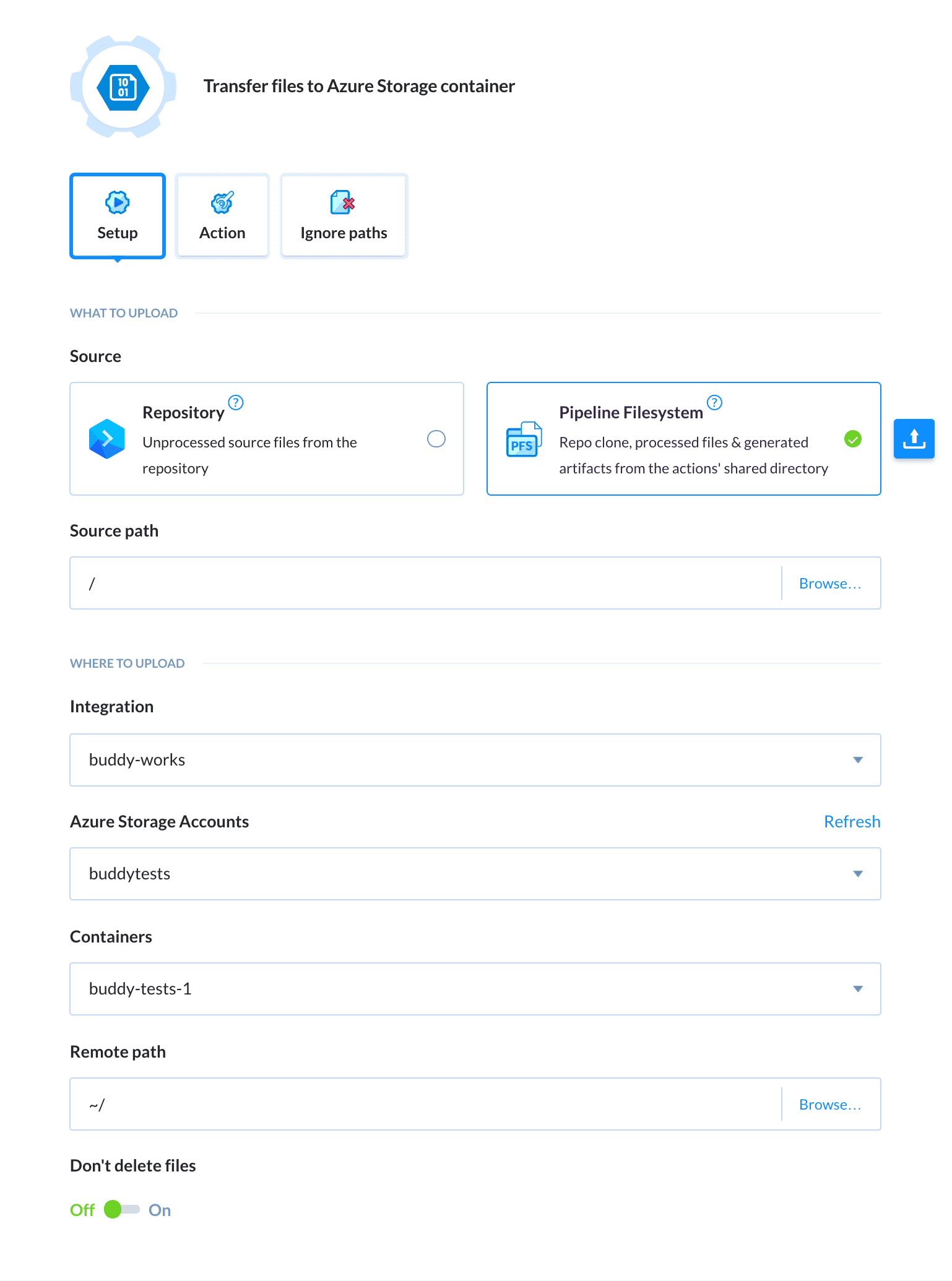The image is a cropped screenshot from a "Transfer Files to Azure Storage Container" page. At the top, the Azure Files logo is prominently displayed, followed by the title, "Transfer Files to Azure Storage Container," in bold black text. Below the title, there are three navigational boxes labeled "Setup," "Action," and "Ignore Paths," with the "Setup" option currently selected.

Under the "Setup" title, in small blue letters, there’s a hyperlink reading "what to upload." The section is categorized under "Source," and features two horizontally aligned boxes: the first labelled "Repository" with a descriptive paragraph below it and the second, labeled "Pipeline File System," which is currently selected. Adjacent to "Pipeline File System" is an upload icon.

Continuing down, the next label reads "Source Path," with a corresponding text box positioned below it. To the right of this text box is a "Browse" button.

Further down, another blue hyperlink titled "where to upload" can be seen. Below this, the section is categorized under "Integration" and includes several drop-down options: "Azure Storage Accounts," "Containers," and "Remote Path," each accompanied by its respective drop-down box. Next to the "Remote Path" field, there is another "Browse" button. At the bottom, there is an option labeled "Don't Delete Files," with an adjacent toggle switch that is currently set to "Off."